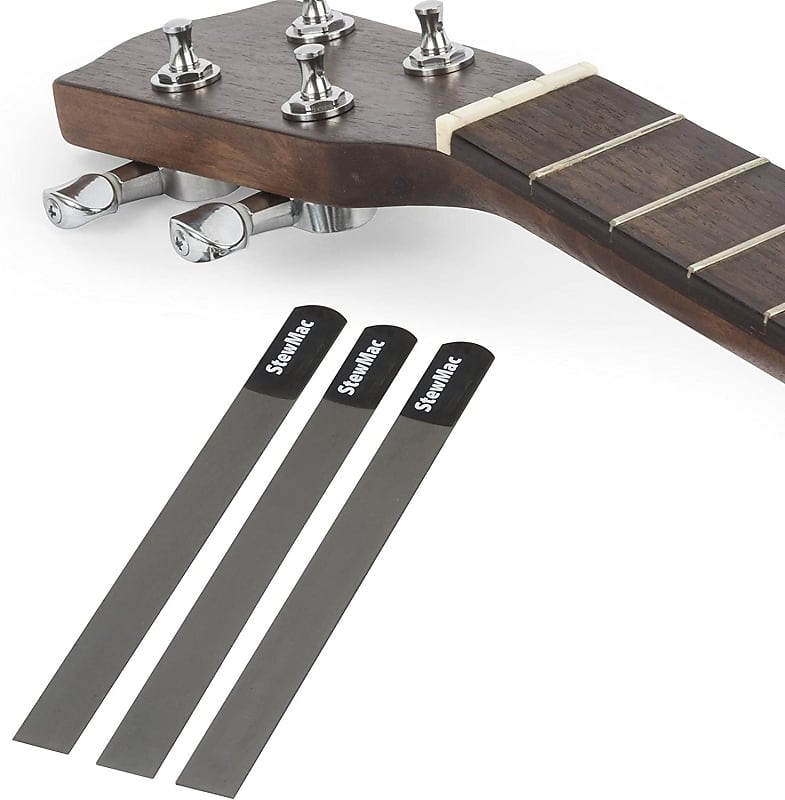This is a detailed close-up photograph of a musical instrument, likely a bass guitar or possibly a guitar, captured against a smooth, white background, suggesting it is a product picture. In the top right corner of the image, you see the headstock of the instrument, made of dark brown wood with silver and white accents. This section displays four silver tuning pegs, which are i.e., knobs used for adjusting the tension of the strings, although the strings are not visible in the photo. The lighting appears to come from the side, softly illuminating the wood and metal components without harsh reflections.

Below the headstock, aligned neatly on the white backdrop, are three identical nut slotting files that are grey and black in color. Each file has a black coating at the end, emblazoned with the brand name "Stew Mac" (S-T-E-W-M-A-C). The files are meticulously arranged, enhancing the advertisement's aesthetic appeal. This well-composed product shot highlights the craftsmanship and clear detailing of both the instrument and the files, making it an effective marketing image.